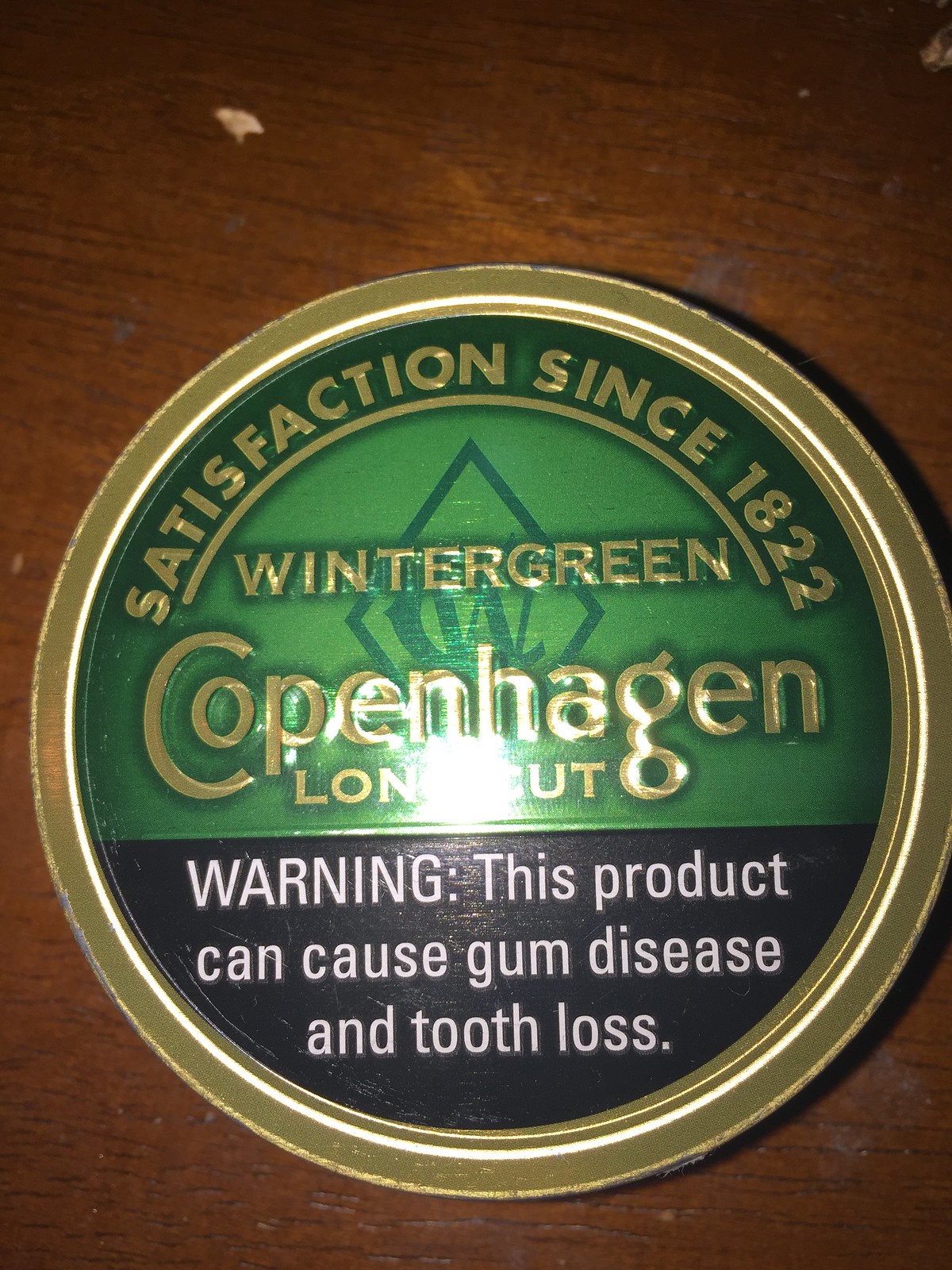The vertical photograph is a closely-cropped overhead shot of a can of chewing tobacco placed on a wooden tabletop with visible wood grain patterns. The circular can, positioned near the edge of the frame with part of it slightly cut off, features a gold outer rim and a predominantly green label divided into two sections. The upper semicircle of the label is green and displays the text, "Satisfaction since 1823," along with the brand name "Copenhagen" and the partially obscured word "LONGCUT" due to a reflection. The lower part of the label is black, with a prominent white warning that reads, "Warning: This product can cause gum disease and tooth loss." The overall composition and details suggest that the product is Copenhagen Wintergreen chewing tobacco.